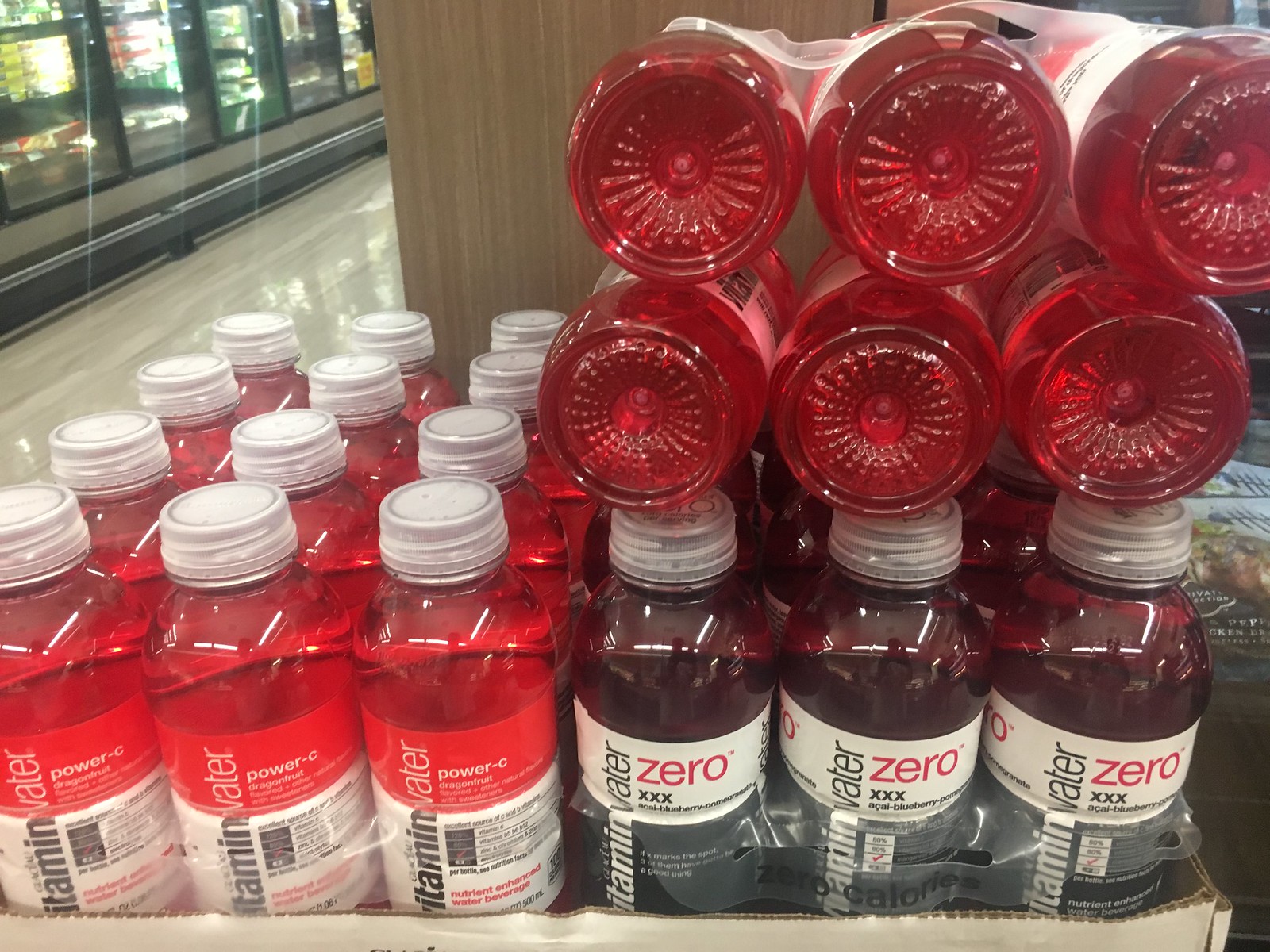The photo is taken in a grocery store and depicts an end-of-aisle display of Vitamin Water bottles. The setup includes a white cardboard tub that contains two main types of flavored water. Positioned on the left side are 12 bottles of a red liquid arranged in three rows of four. These bottles feature a distinctive label: the bottom half is white, the upper section is red, and the text "Vitamin Water" is prominently displayed. Furthermore, these bottles are labeled "Power C." 

On the right side of the display, there are bottles with a darker red or purple hue. These are also arranged in rows, and there are a few additional bottles of the red Vitamin Water laid horizontally on top. The darker bottles have a unique label with a black bottom section and a white top section that says "Zero" in red, followed by three X's underneath.

The display is situated near the corner of the store, adjacent to refrigerated or freezer compartments visible in the upper left of the image. The area features a wood-grain shelf immediately behind the display, and the white floor reflects light, adding to the store’s bright ambiance.